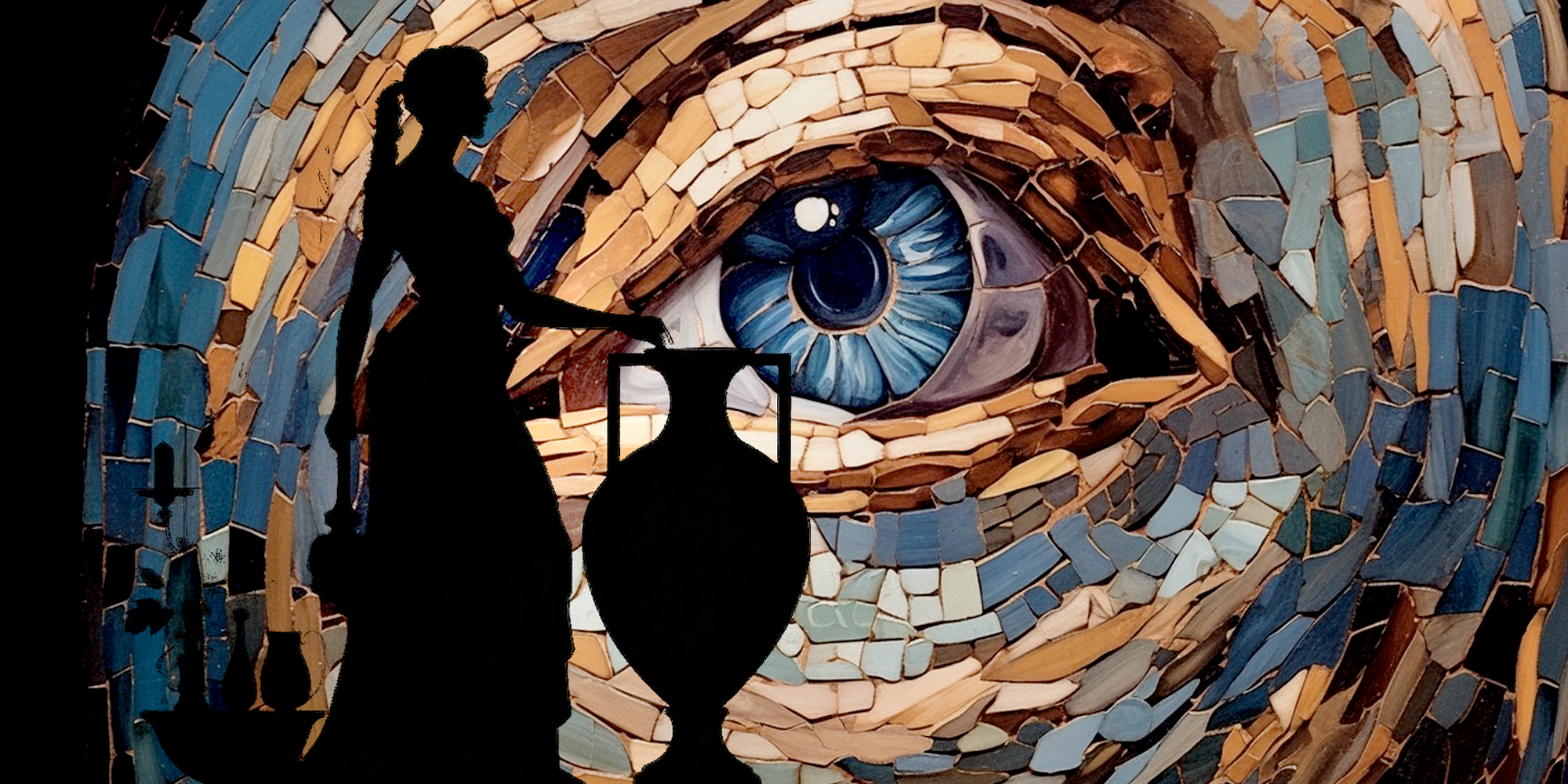The image features a striking animated graphic, characterized by a detailed mosaic on the back wall composed of small, multicolored tiles. These tiles, varying in shades of blue, white, brown, and gold, intricately form the eye area of a face. Prominently in the center, a blue eye with a black pupil is depicted amidst the mosaic. On the middle left, the shadowy silhouette of a woman with a long braid is seen, her gaze directed towards the eye. Her silhouette is black, as is the tall vase or jug she touches with one hand, adding to the scene's abstract allure. The jug, resembling the shape of a spade, subtly accentuated by two handles, completes this vivid and artistic tableau.